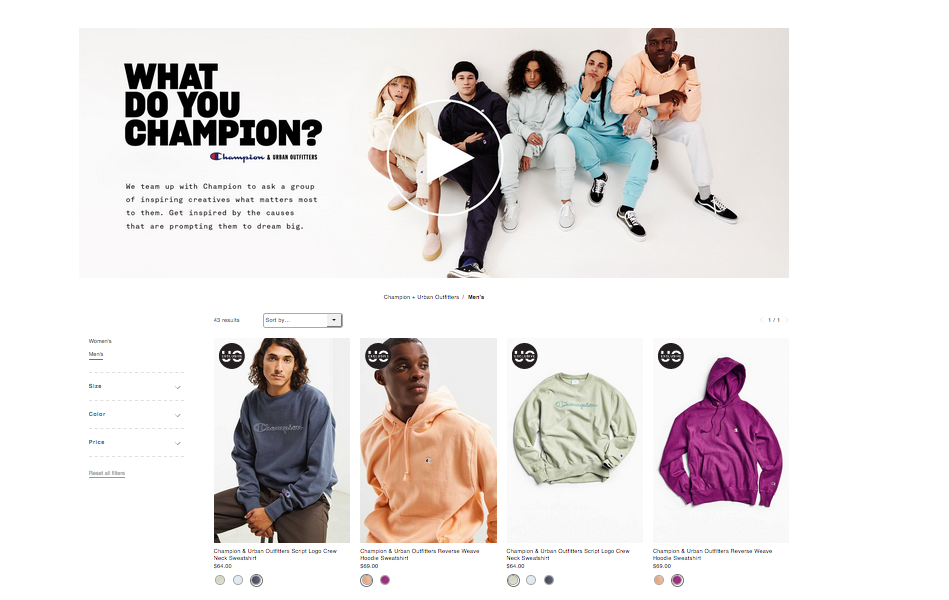**Website Shopping Page Screenshot**

At the top of the webpage, there is a rectangular photograph showcasing five individuals dressed in coordinated sweatpants and sweatshirts, seated in a row against a beige background. The group gazes ambivalently at the camera. Superimposed centrally on the image is a white outlined circle with a white triangle inside, pointing to the right, indicating a play button.

In the top left corner of the image, bold black text spans three lines: "WHAT DO YOU CHAMPION?" Down and to the right, there is a stylized logo with the word "CHAMPIONS" in blue. The initial "C" is considerably larger and contains a red blob within its left interior. Adjacent to this logo, there is black text in all caps: "URBAN OUTFITTERS."

Below the image, a four-line paragraph in black text reads:
"WE TEAM UP WITH CHAMPION TO ASK A GROUP OF INSPIRING CREATIVES WHAT MATTERS MOST TO THEM. GET INSPIRED BY THE CAUSES THAT ARE PROMPTING THEM TO DREAM BIG."

Continuing down, the main body of the webpage features a white background. At the center top, small black text reads "CHAMPIONS" followed by an arrow pointing right, and "URBAN OUTFITTERS / MEN'S," with "MEN'S" bolded.

On the left side, there is a sidebar with a white background. At the top left of this sidebar, small black text reads "WOMEN'S." Directly underneath, "MEN'S" appears, underlined in black. A dotted light gray line separates these sections, with various options listed beneath.